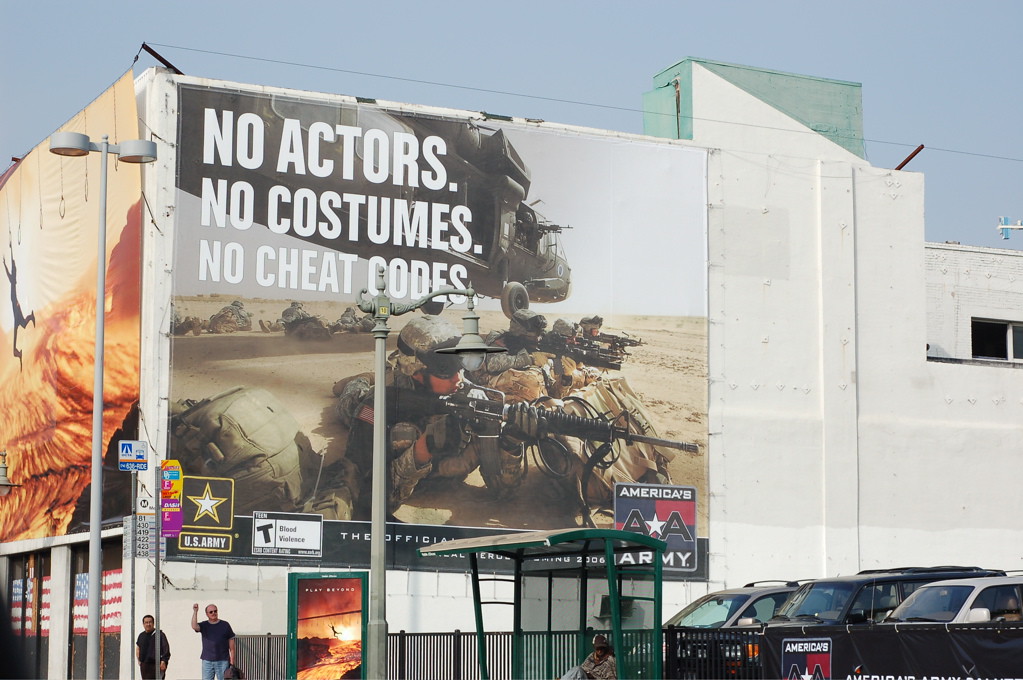The image depicts a large advertisement for the U.S. Army's game, America's Army, prominently displayed on the side of a white building. The ad, titled "No actors, no costumes, no cheat codes," features a detailed portrayal of army soldiers equipped with camouflage gear, goggles, and guns, resting on a desert-like terrain. Above the soldiers and the slogan, a helicopter hovers in a grayish sky, adding to the realistic military setting.

Adjacent to this, on the front of the building, another advertisement shows the silhouette of a man navigating a series of suspended rings, reminiscent of obstacles in a jungle gym, set in a desert environment. The building is surrounded by a green fence, and nearby, several vehicles and people are visible, including someone sitting at a bus stop bench with bus numbers displayed. The ad is rated T for Teen by the ESRB, indicating it contains blood and violence. The scene captures the immersive and gritty appeal of the America's Army game, developed and sponsored by the U.S. Army, reflecting a mid-2000s release era.